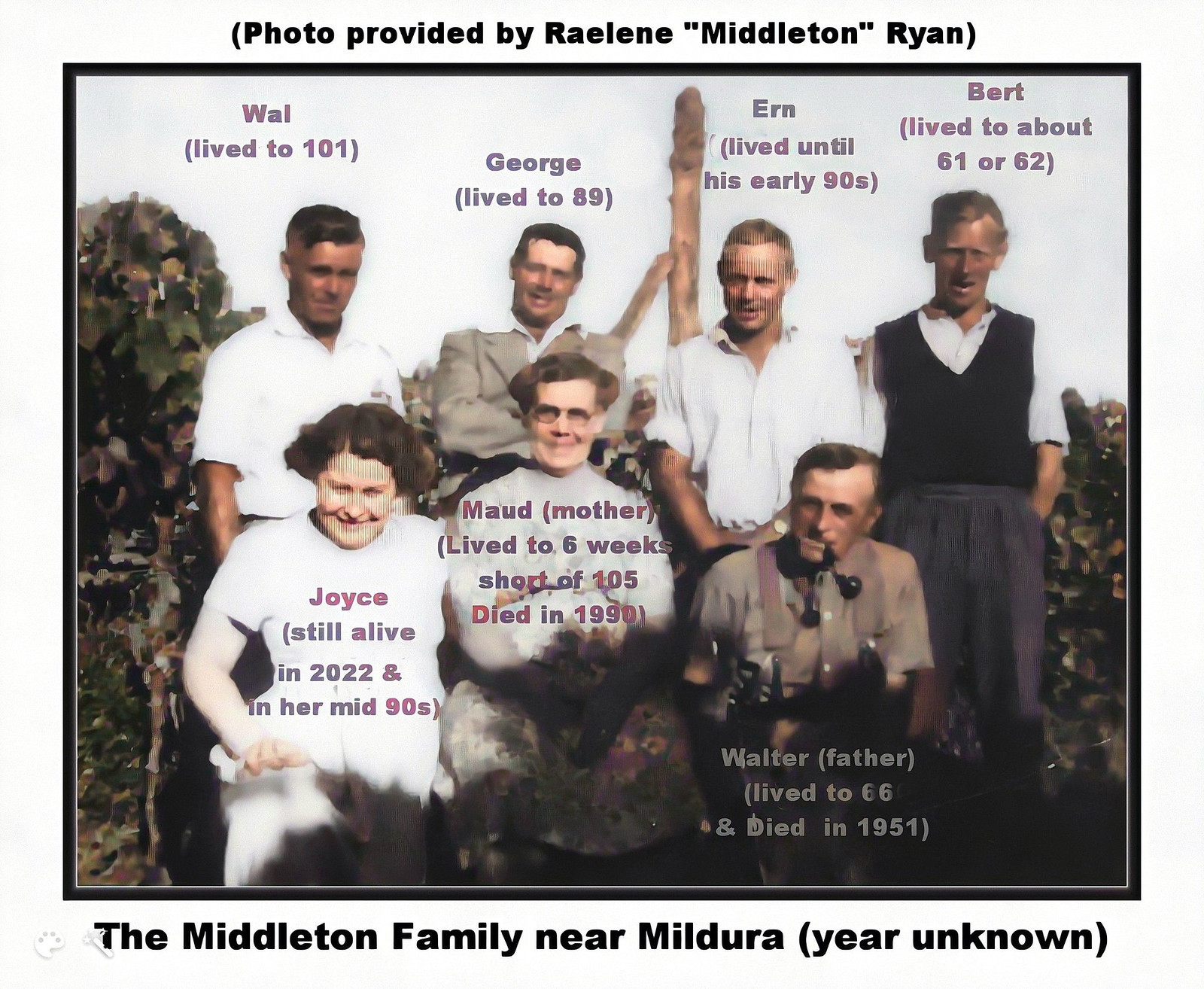A remarkable vintage photograph capturing the Middleton family near Mildura, its year of capture unknown. Provided by Raylene 'Middleton' Ryan, the image features seven elderly family members. The back row comprises the men: Wall, who lived to 101, George, who reached 89, Earn, who lived into his early 90s, and Bert, who passed at about 61 or 62. Sitting at the front are Joyce, who was still alive in 2022 and in her mid-90s, alongside her parents, Maud and Walter. Maud, the matriarch, almost reached 105 years, passing away in 1990, while Walter, the father, lived until 66, passing in 1951. Their attire, reminiscent of the 60s or early 70s, and the image's aged quality suggest a classic, possibly 70s or 80s photo, set in a rustic outdoor setting, likely a vineyard or the family yard, adding to the timeless and enduring appeal of this family legacy.